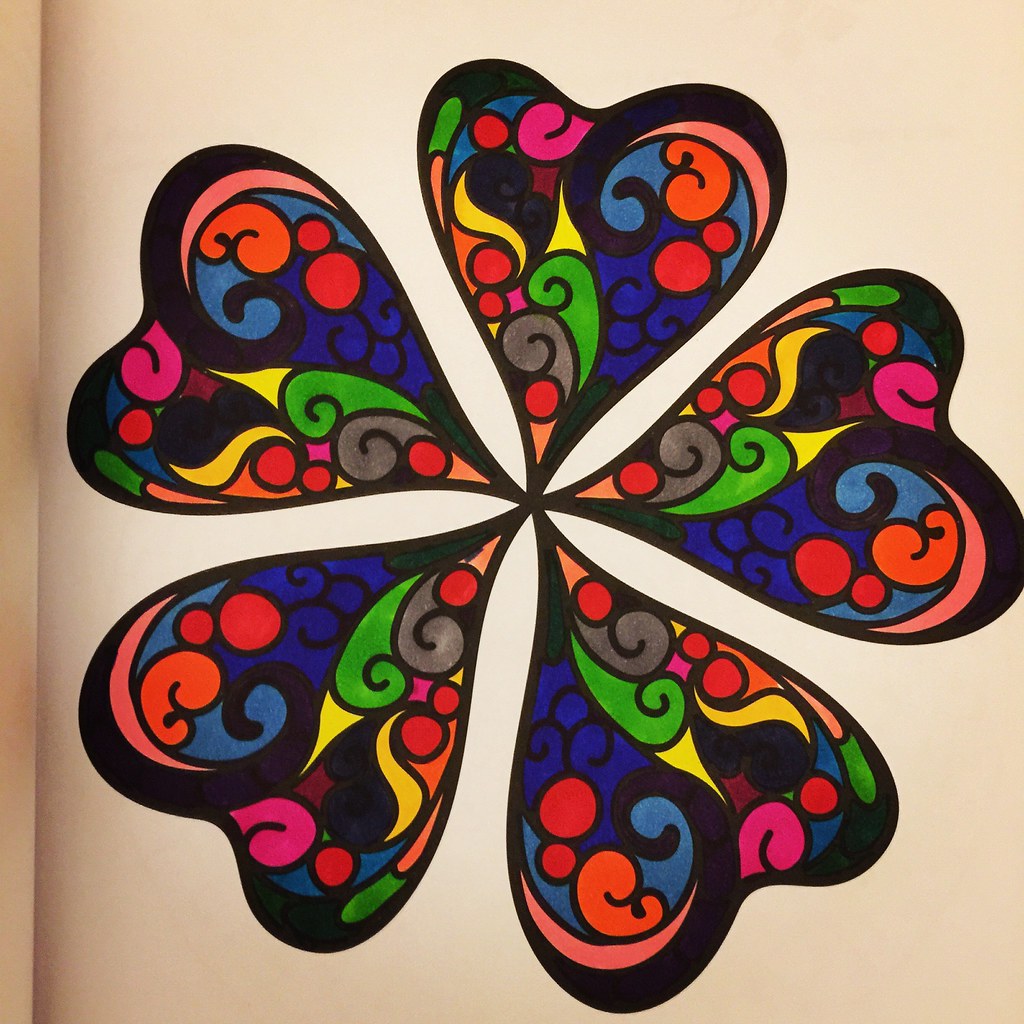This vibrant image, set against a pale pink background, appears to be reminiscent of an adult coloring book illustration. The backdrop is outlined in dark black ink, creating intricate sections meticulously filled in with marker colors. At the center of the composition is a five-petaled flower, devoid of a central stigma, with petals converging elegantly at the heart. Each petal mirrors the others, featuring a harmonious gradient that transitions through a spectrum of colors: medium green, pink, red, royal blue, yellow, light purple, peach, lighter blue, and darker blue. The meticulous coloring technique used gives the image a polished, vibrant quality, showcasing the artist's precision and attention to detail.